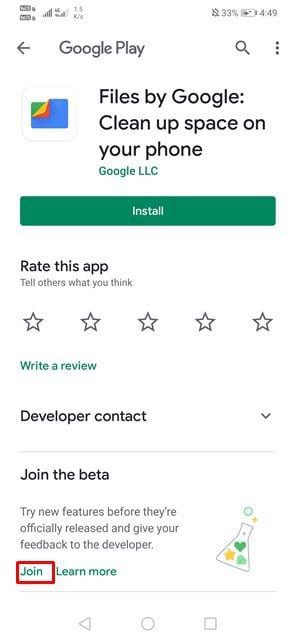The image depicts a screenshot from an Android phone showcasing how to join the beta program for the "Files by Google" app via the Google Play Store. The phone's battery level is at 33%, and it is currently plugged in. The screenshot highlights the app's page, specifically for "Files by Google - Clean up space on your phone" developed by Google LLC. 

In the upper section, the icon and title of the app are displayed prominently, alongside buttons to "Install" and "Rate the app." The page also indicates the app's current star rating and offers the option to write a review. Below these elements, there's a "Developer contact" option providing a channel for users to get in touch with the app's support team.

A significant focus of the image is the "Join the Beta" section, which invites users to "Try new features before they're officially released and give your feedback to the developer." The "Join" button is highlighted with a red box, drawing attention to the process of joining the beta program. Additional details about the beta program are indicated through a "Learn more" link. At the bottom of the screen, the typical navigation buttons of an Android device are visible.